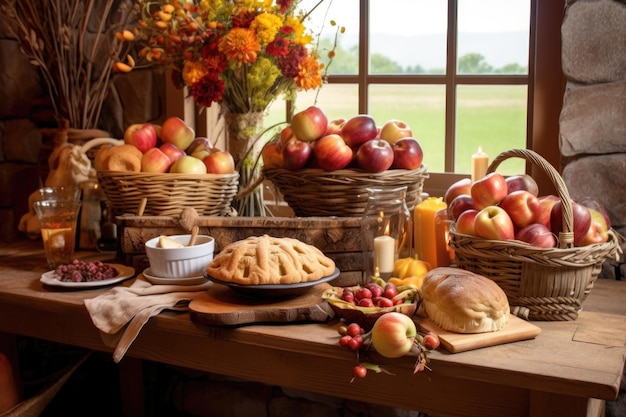The image depicts a rustic, autumnal tablescape set within a cozy stone-walled room. A large, wooden table is generously adorned with an array of food items that evoke warmth and abundance. The focal point includes three woven baskets brimming with apples, accompanied by a loose apple on the wooden surface, a small bowl of cherries, a loaf of bread on a chopping board, and a lattice-topped pie suggesting the relaxed comfort of a countryside setting. There are also floral arrangements in vases adding a touch of natural beauty. Scattered on the table are candles, various drinks, and additional dishes, including a white ceramic dish containing an indeterminate item and some sort of berry. The warm, inviting earth tones of yellows, oranges, reds, and browns dominate the color palette, with hints of green and a pocket of chartreuse adding contrast. In the background, a window with eight panes framed by wooden slats offers a glimpse of a serene green landscape, further enhancing the bucolic charm of the scene. The overall atmosphere is captured with a sepia-like tone, creating an almost painted or digitally rendered quality to the image, imbuing it with a quaint, slightly surreal feel.